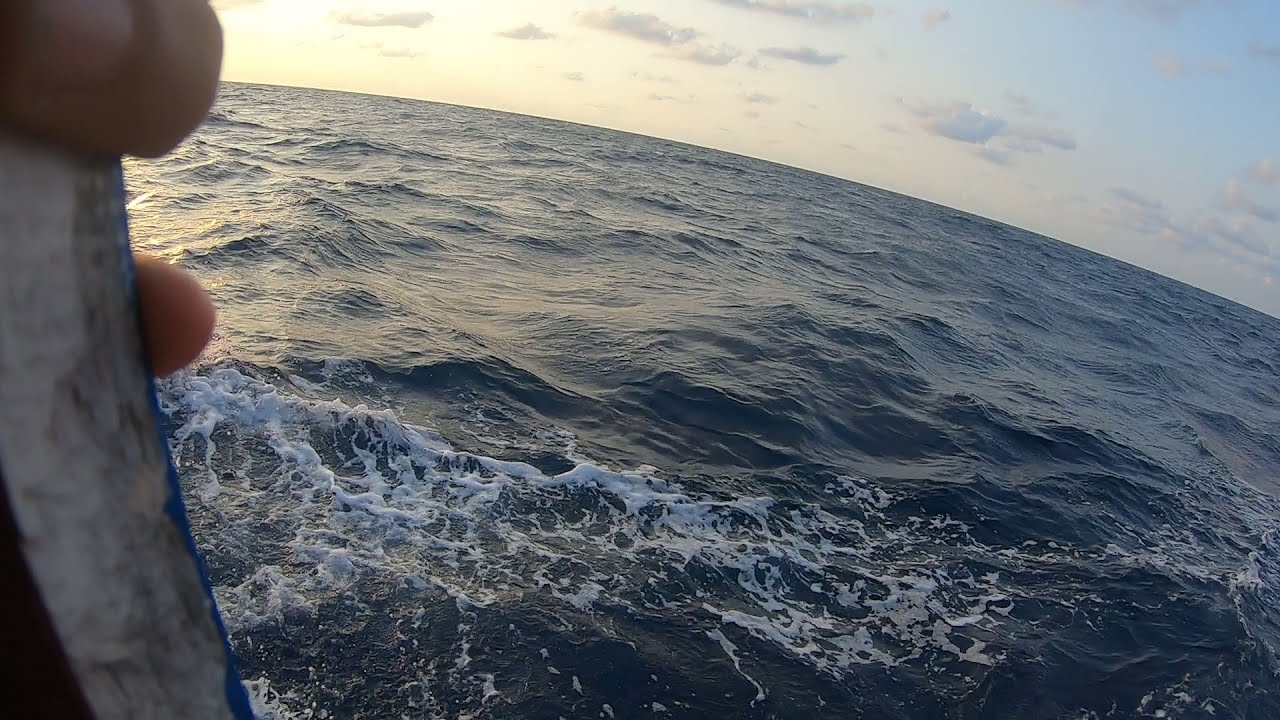The image depicts a vast ocean scene with the majority of the frame occupied by dark, slightly wavy water interspersed with patches of white sea foam, particularly towards the bottom and left. The horizon curves gently from the top left to the middle right, accentuating the curvature of the Earth. The sky above transitions from a bright, almost glowing yellowish-pink on the left, suggesting the setting sun, to a serene blue with sparse clouds on the right. In the foreground, two fingers are visible on the left edge of the picture, gripping a flat, grayish object that appears to have traces of blue paint. The overall impression is one of serene beauty, capturing the vastness of the ocean and the subtle hues of the sky at sunset.